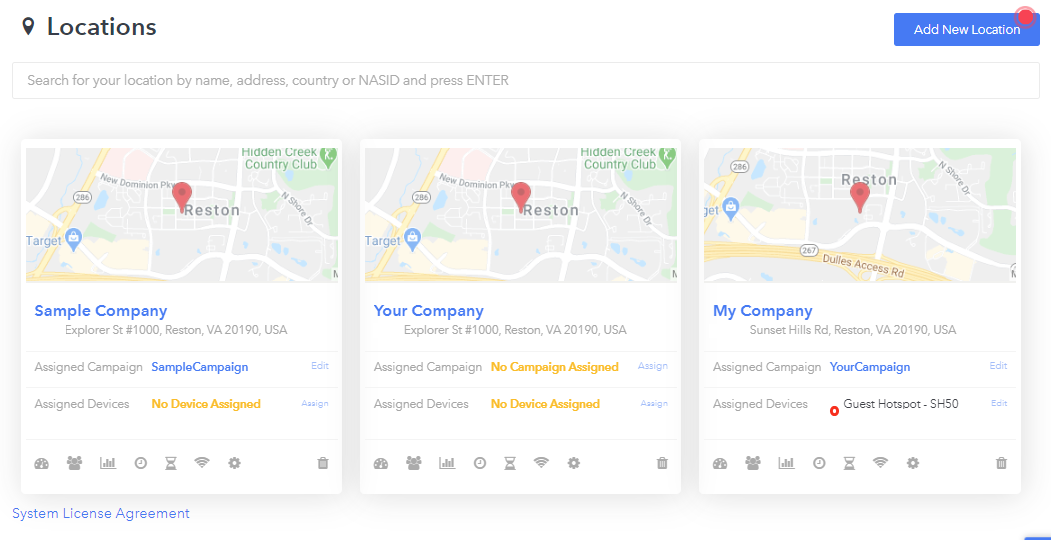In the upper left corner of the image, the word "Locations" is prominently displayed. On the far right, inside a blue rectangle, there's a label that reads "Add New Location," accompanied by a small red dot. Positioned below is an open search bar with the placeholder text "Search for your location by name, address, country, or NAZID and press enter."

To the left, a section of the image from Google Maps is visible, featuring Hidden Creek Country Club indicated by a green map marker. At the center, a red map marker is labeled "Reston," which is clearly spelled out (R-E-S-T-O-N). To the far left, next to a blue marker, the word "Target" is noted. Below this, the text "Sample Company" appears in blue.

On the right side, once again, the red map marker and the word "Reston" are repeated. Below this, it specifies "Your Company, Explorer Street number 1000, Reston, Virginia, 20190, USA." Adjacent to this, the same map is again visible at the top, but with the addition of a yellow diagonal or horizontal line labeled "Dulles Success Road." Below this line, in blue text, it lists "My Company" and "Assign Devices" followed by "Guest Hotspot SH50."